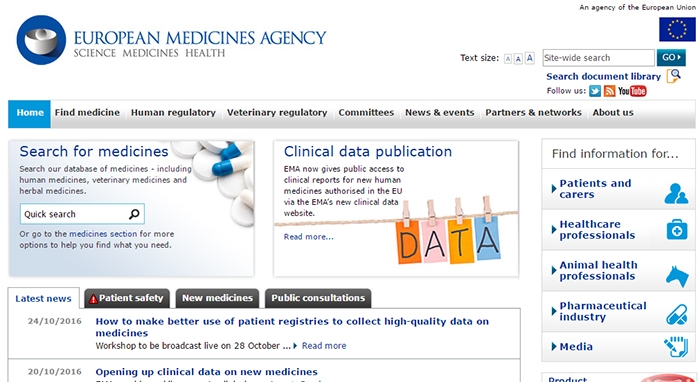The image showcases a detailed view of a webpage belonging to the European Medicines Agency, prominently titled "European Medicines Agency: Science Medicines Health." The page is primarily composed of a white background with blue text and various tabs for navigation. The header includes a circular white cup icon set against a blue background.

Highlighted in blue is the "Homepage" tab, indicating it is the currently active section. Other tabs available for navigation include "Find Medicine," "Human Regulatory," "Veterinarian Regulatory," "Committees," "News and Events," "Partners and Networks," and "About Us." There is also a search box located on the page, along with social media follow options for Twitter and YouTube.

A section titled "Find Information for" is present, catering to different audiences such as Patients and Caregivers, Healthcare Professionals, Animal Health Professionals, the Pharmaceutical Industry, and Media. The website features a "Latest News" section with an entry dated 24-10-2016, headlined "How to Make Better Use of Patient Registries to Collect High-Quality Data on Medicines."

In addition, there are tabs for "Search for Medicines" and "Clinical Data Publication." The page includes various graphics: an image of white pills and another featuring a collection of cards that spell out the word "Data."